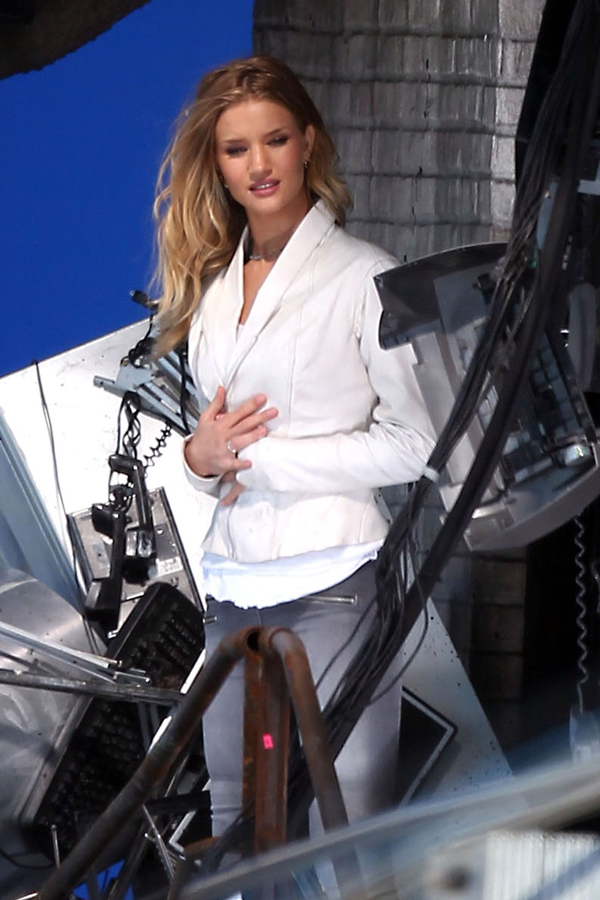In this detailed photograph, a woman with long, flowy, wavy, dirty blonde hair that lightens towards the edges is standing in an indoor setting. She has brown hair part down the middle and wears thick eyeshadows and lipstick, giving her a model-like appearance. She is smiling and dressed in a white suit jacket over a white t-shirt, paired with gray, fitted pants that feature zipper pockets. Her hands are interlaced over her stomach, and a ring adorns the third finger of her right hand. 

The background is a mix of settings with a blue wall visible on one side and a brown wall on the other, creating a visually contrasting backdrop. To her side, there is a grayish pillar constructed of thick concrete bricks. Surrounding her is an array of machinery and various objects, including lamps and cameras, interconnected by a network of wires. This intricate setup suggests that the photograph was taken in a photoshoot setting, with the woman posing amidst the equipment. The image is taken in a portrait orientation.